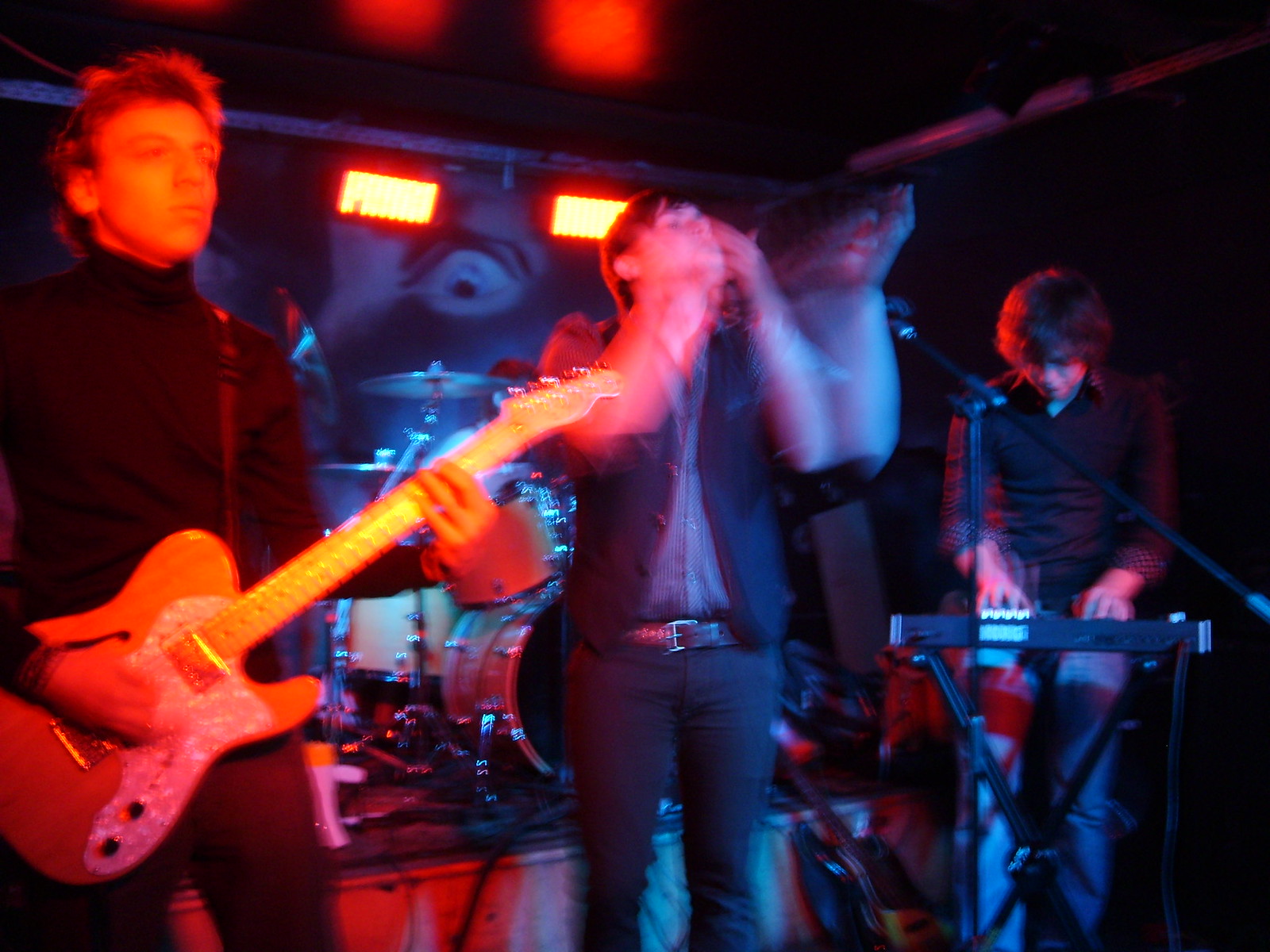This indoor concert photograph captures a dynamic and slightly blurred image of a three-man band performing under dim, atmospheric lighting. Centered in the frame is the lead singer, who appears to be playing a harmonica. He is dressed in a black suit with a brown belt, his movements rendered in a stop-motion-like blur, suggesting dynamic action. To the left, a guitarist in a dark suit plays an electric guitar, his face and hands glowing orange due to the distinctive stage lighting. On the right, a young white man with a microphone attached to his head bends over a synthesizer mounted on a stand, his attire dark and most likely comprising a shirt and jeans. The background reveals a set of drums positioned on a raised platform and illuminated by spotlights, with two prominent orange lights providing additional stage ambiance. Although the lighting and movement obscure finer details, there seems to be a name, potentially "Yamaha," faintly visible on the keyboard.